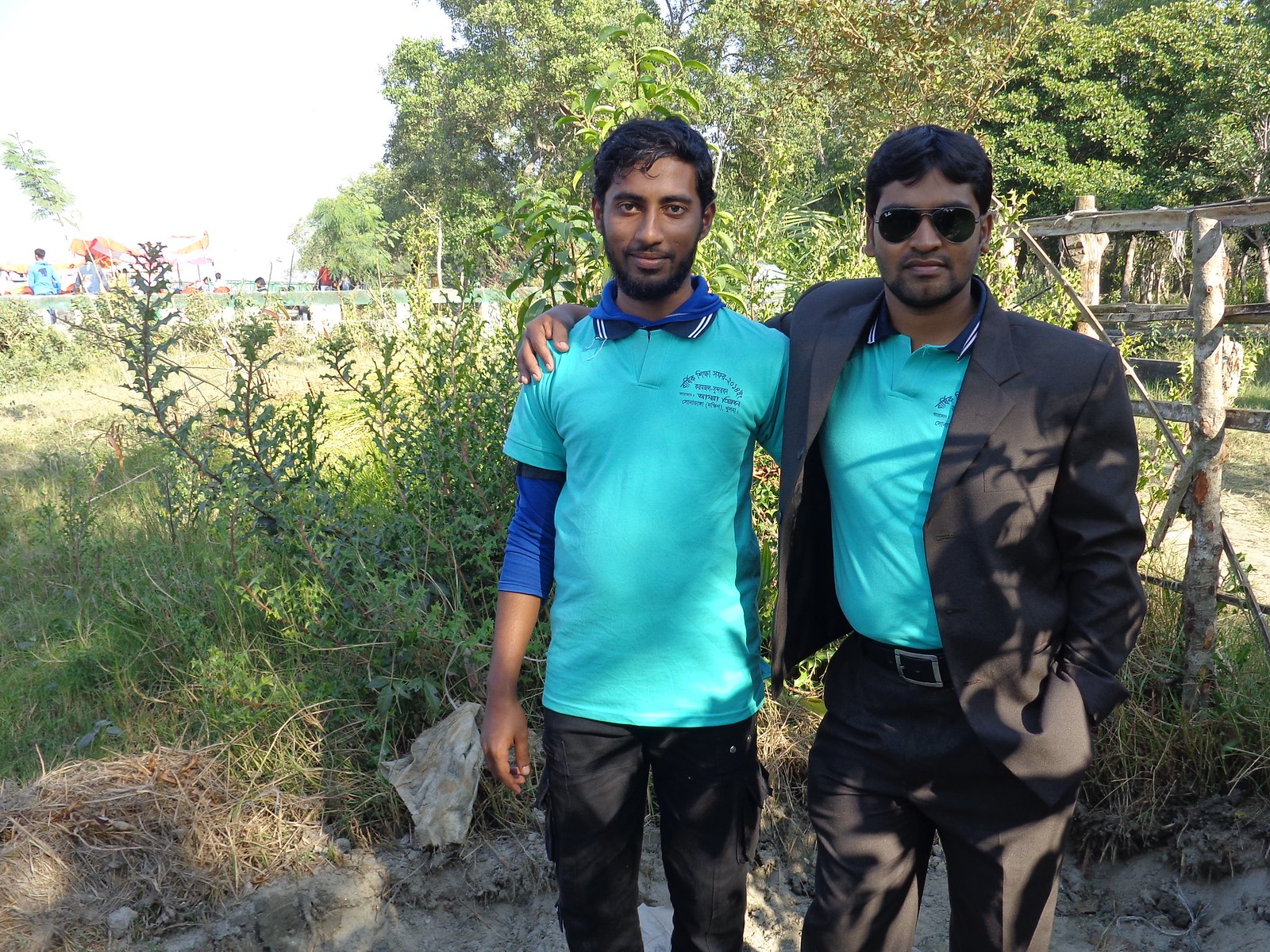The photograph captures an outdoor scene on a sunny day with intermittent clouds. Two gentlemen, who seem to be of Indian or Pakistani descent, are the focus of the image. Standing in a verdant and somewhat overgrown grassy area with extensive tree cover, they both appear to be enjoying the natural surroundings, partially shaded by the trees. Behind them is an old, rusted walkway and what appears to be a low wall, beyond which there are faint figures of people and possibly water in the far background. 

The man at the center of the image is wearing a short-sleeved aqua blue T-shirt over a long-sleeved dark blue collared shirt and black slacks. He has a mustache, finely trimmed beard, and a subtle smile while looking directly at the camera. The man on his right, who is slightly heavier set with broader shoulders, sports similar attire with the addition of a gray dress coat and dark aviator sunglasses. He has his right arm around the shoulders of the man beside him. Both men have black hair and brown skin, indicating their likely Middle Eastern or South Asian heritage.

The image is rectangular, roughly measuring four by six inches, and it is framed to show the men from about the knees up on the right side of the picture. The background includes green shrubs, trees, and a wooden fence to the right, offering a rustic, unkempt charm. Overall, the scene conveys a casual yet endearing moment shared between the two friends amidst a lush, natural landscape.